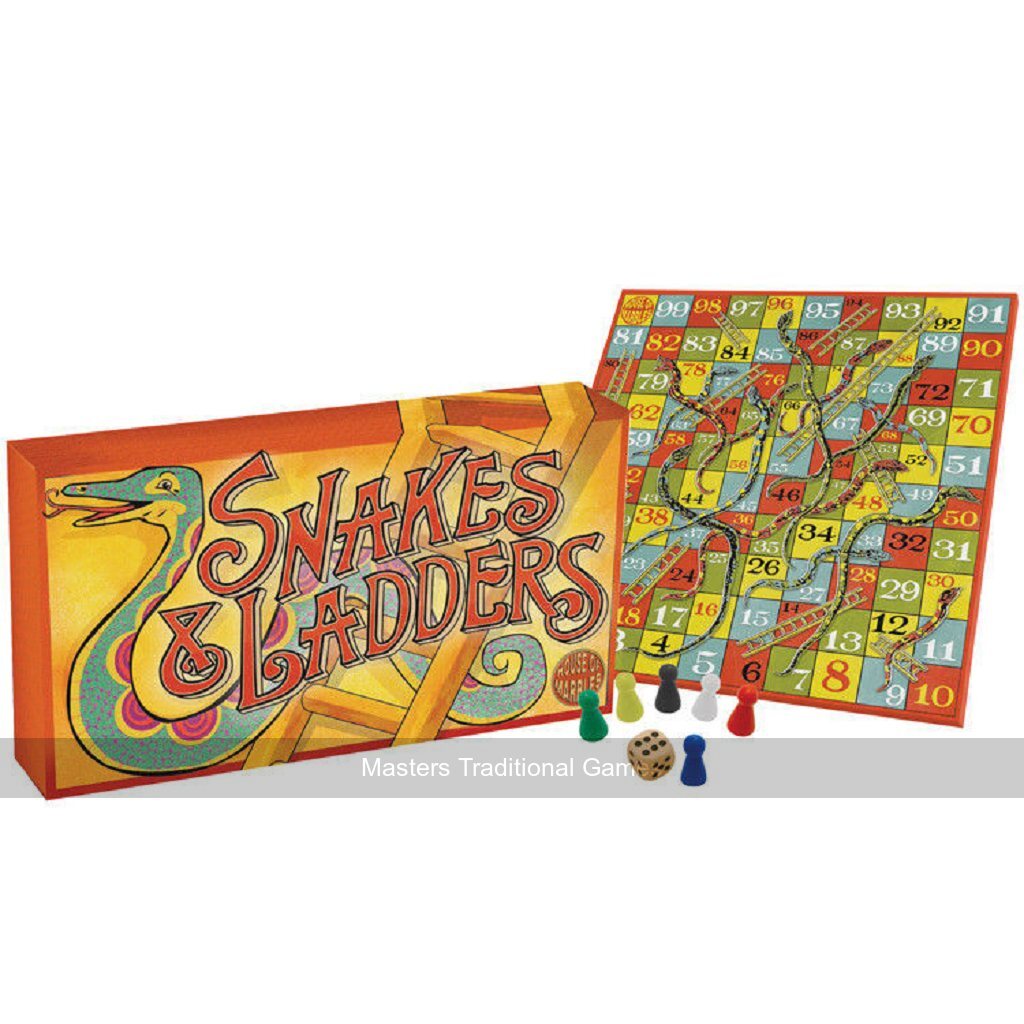The image depicts a vibrant board game called Snakes and Ladders. On the left side, the box showcases an animated, colorful design. The box features an orange border on the top and left sides, with a yellow background. Prominently displayed in red lettering is the game's title, "Snakes and Ladders." A teal snake with yellow accents and pink and purple stripes winds its way around the box. The snake's head points left with its mouth open, its body looping behind the title before curling to a point on the right. A wooden-colored ladder is positioned behind the snake.

On the right side is the game board itself, comprising a grid pattern of squares in various colors: blue, red, and green, each numbered sequentially. Below the board are the playing pieces, resembling tiny thimbles, available in green, yellow, black, blue, white, and red. A single die showing the number six is also present. At the very bottom, a light gray bar with white text reads, "Master's Traditional Game."